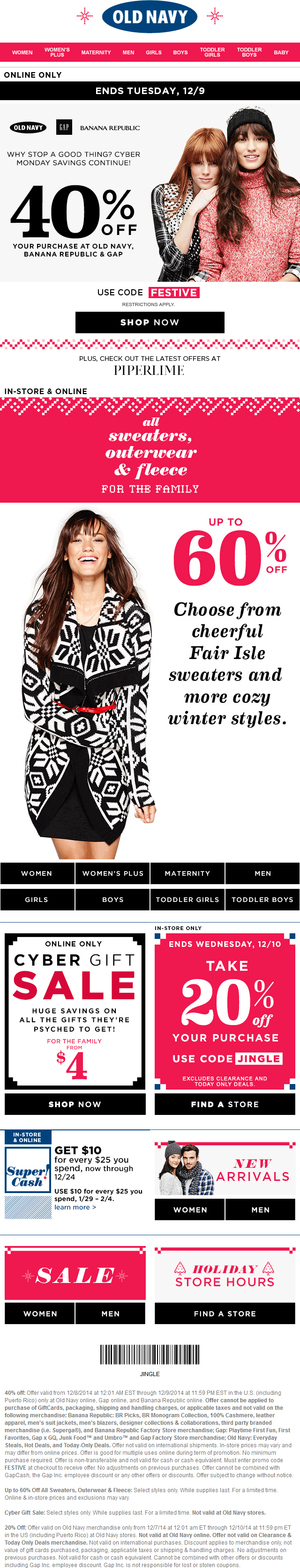This old Navy advertisement appears to be stretched out, which has reduced the resolution and clarity. At the top of the image, the iconic Old Navy logo is displayed within a blue circle, flanked by two stars and situated in a reddish-pink navigation bar that's hard to decipher due to the stretching. A black line under the logo reads “Tuesday 12/9,” with “Online Only” noted above it, though some text is illegible.

The main promotion highlights a 40% off deal and features two female models: one in a black sweater and the other in a pink sweater. The phrase “Use Code FESTIVE” is prominently displayed alongside a black “Shop Now” button. A stylish diagonal line separates this section from the lower portion of the ad.

In the lower section, a red banner announces sweaters, outerwear, and fleece items with discounts of up to 60% off. A large red caption on a white background reads, “Choose from cheerful Fair Isle sweaters and more cozy winter styles.” 

To the left, a woman in a black-and-white festive sweater with brown hair and fair skin is featured, with black navigation buttons below her image. Beneath this are two online-only advertisements promoting a “Cyber Gift Sale” with 20% off coupons. Each ad has a “Shop Now” button on the left and a “Find a Store” button on the right, alongside more coupon details.

At the very bottom, a barcode and additional information are present, although they are difficult to read due to the image's poor resolution.